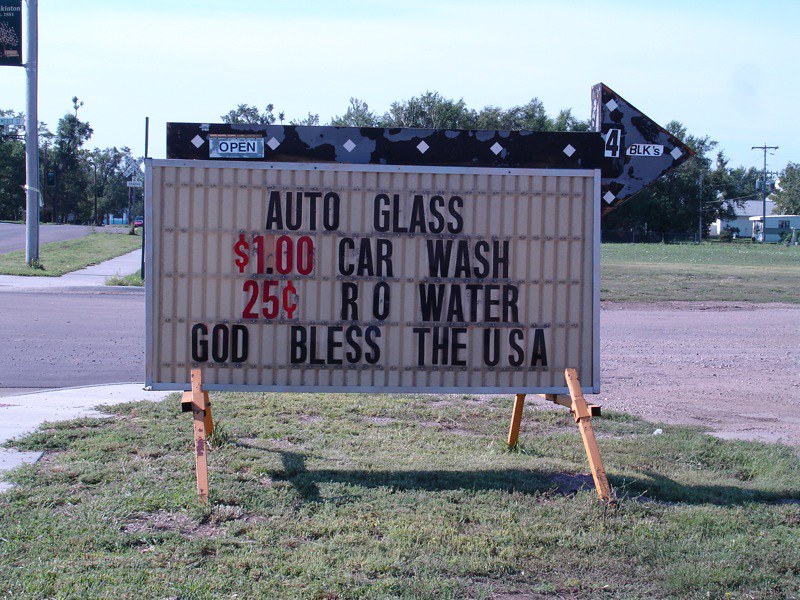This outdoor photograph captures a vibrant scene along a roadside, framed by a clear blue sky. The focal point is a sign situated on a patch of mostly green grass, which is held up by four wooden supports. The sign prominently features a large black arrow with blue spots pointing to the right, marked “OPEN” along the arrow's shaft and “4 BLKS,” directing viewers to a nearby business.

The sign displays several messages in alternating red and black letters: “Auto Glass,” “$1 Car Wash,” “25¢ RO Water,” and “God Bless the USA.” Surrounding this sign, the scene shows a street running left to right across the foreground and another street extending down on the left side, where a red car is approaching. On the opposite side of the road, there is a sidewalk adjacent to a grassy area.

In the background, a neighborhood is visible with houses, trees, and power lines. A streetlight stands on a corner, and there are additional elements such as a banner on another pole and what appear to be caravans or trailers towards the top right, amidst more trees and power poles. The entire scene gives a sense of a small, well-settled community touched by a sunny day.